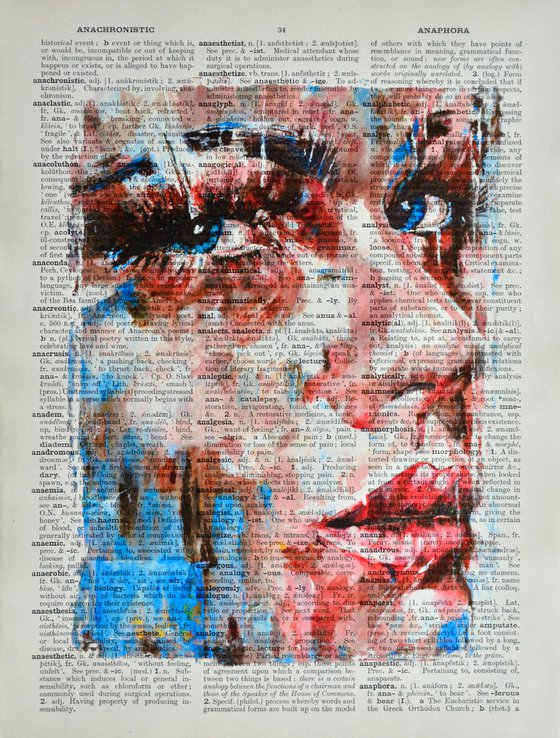The image features a page from an old dictionary or encyclopedia, designated as page number 34, containing black text definitions of words beginning with the letter 'A', including "anachronistic" and "anaphora." Over this textual background, a vibrant, modern watercolor painting of a woman's face stands out. The woman, who appears to have a pale complexion with varying shades of red and blue, gazes directly at the viewer with striking blue eyes. Her head is slightly turned to the right, but her eyes are notably focused forward, creating an engaging and somewhat enigmatic look. The face outlines and details, such as the slit eyebrows and full lips adorned with lipstick, are primarily highlighted with blue, giving the painting a unique, modern, and dynamic appearance against the grayscale background of the dictionary page.